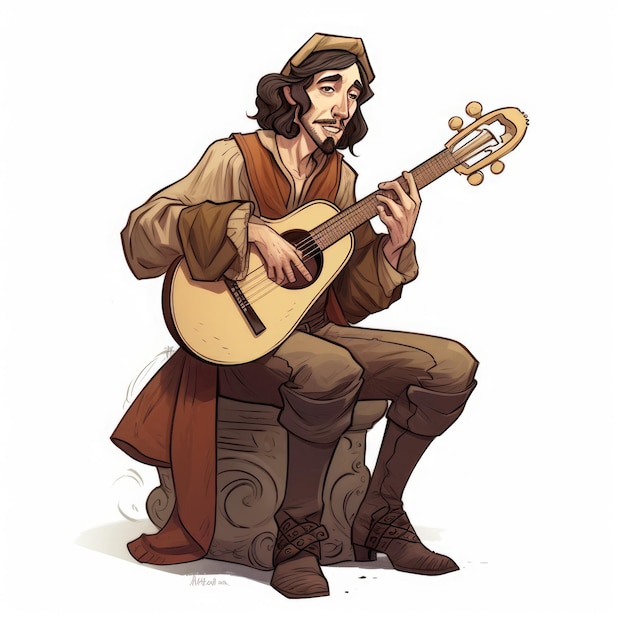This detailed animated illustration features a somber-looking man sitting on a stone bench, playing a guitar, set against a solid white background. The man is oriented towards the right, with his mouth open as if singing or speaking. His appearance is reminiscent of a renaissance fair minstrel, characterized by long, slightly curly dark brown hair that reaches just above his shoulders, a thin brown mustache, and a triangular chin adorned with a goatee. His expressive face is completed with thick brown eyebrows and droopy brown eyes.

He is dressed in an earth-toned outfit consisting of a light brown shirt with baggy sleeves, a dark brown vest, and a tan hat that adds to his medieval aesthetic. The vest appears to flow down his back, resembling a cape that drapes over the bench and onto the floor. He also wears tall brown boots and matching brown pants. The guitar he strums is a light brown, almost yellowish color, with an avocado-shaped body and four strings.

The stone bench he is seated on is a brownish-gray color, adorned with subtle swirled patterns on the sides. The overall composition of the scene, devoid of any border or text and set against a stark white backdrop, emphasizes the detailed, earth-toned attire of the melancholic musician and his musical instrument.